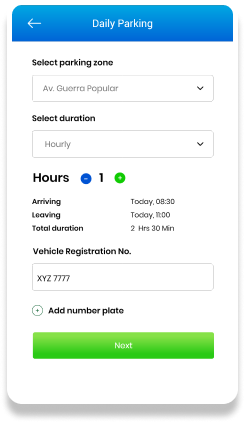The image depicts a digital user interface for Daly Parking, resembling either an overlay purchase screen or a receipt. At the top, there is a blue horizontal bar with white text and a back arrow on the left side, indicating navigation options. Below this, the text "Parking Zone" is displayed in black bold font. Further down, a drop-down menu with a gray background shows "A.V. Guerrero Popular."

The interface prompts the user to "Select Duration," written in blue bold text. This section is set against a white background, continuing the overall white theme of the main background. The duration selection is marked as "Hourly," displayed in gray text. Within this section, bold black text reads "Hours," with a decrement option (minus sign in a blue bubble with white text) on the left and an increment option (plus sign in a green bubble with white text) on the right. Currently, the selected duration is "1 hour."

Additional details include the user's arrival and departure times: "Arriving Today: 08:30" and "Leaving Today: 11:00." The total duration is calculated as "2 hours, 30 minutes," presented in smaller bold text. The categories ("Hours") are on the left, with respective times in dark gray text on the right.

For vehicle registration, an entry box displays the placeholder "XYZ 7777" in gray text. There is an option to "Add Number Plate" with a plus sign next to it. Finally, at the bottom of the interface, a green button labeled "Next" allows the user to proceed, followed by an expanse of white space below.

Overall, the interface combines structured information and user-friendly interactive elements, facilitating a seamless parking selection process.